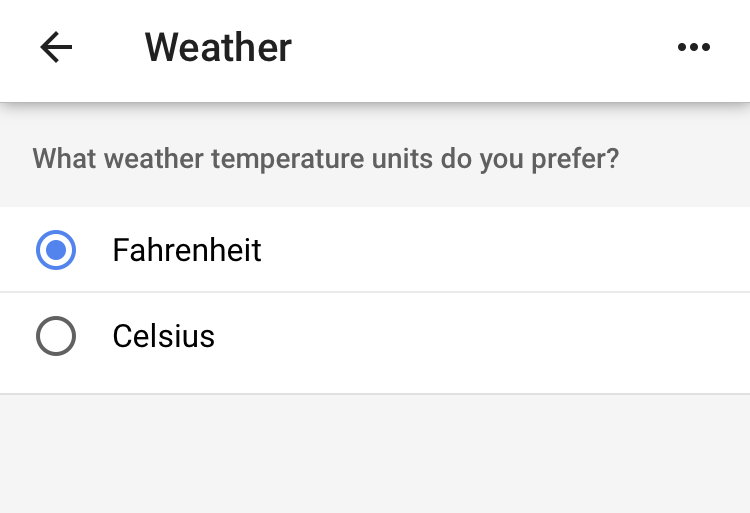In the image, the interface of a weather application is displayed on a predominantly white background. At the top left corner, a black text label reads "Weather," accompanied by a black arrow icon pointing left, symbolizing the 'Back' function. On the top right, three vertically aligned black dots represent the main menu options.

Below the "Weather" label, there is a question in grey text asking, "What weather temperature units do you prefer?" This question rests on a light grey background. Beneath this query, two selectable options for temperature units are presented: "Fahrenheit" and "Celsius." The option "Fahrenheit" is currently selected, indicated by a blue circular checkmark to its left. Both temperature unit labels ("Fahrenheit" and "Celsius") are in black text against a white background. The "Fahrenheit" option appears above the "Celsius" option, providing a clear choice for users to set their preferred temperature unit in the weather app.